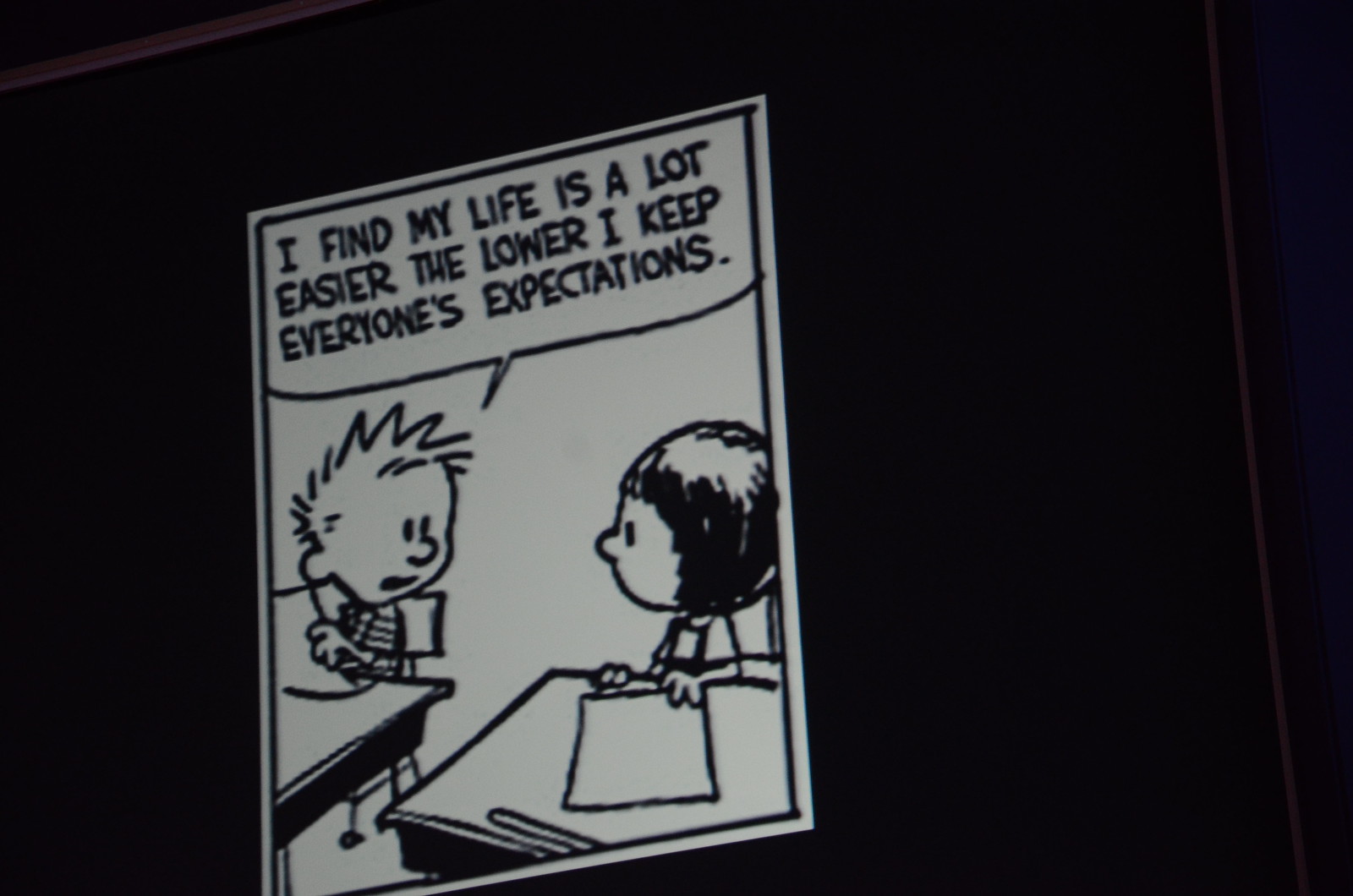The close-up photograph showcases a single, slightly tilted comic panel from Calvin and Hobbes, appearing as if displayed on a dark screen. The panel is white with a thin black border and contains a detailed hand-drawn scene. At the left desk, a boy with spiky hair wearing a black-striped shirt—Calvin—is holding a piece of paper up to his face and looking towards Susie, a girl with dark hair, who is at the right desk. She has a paper laid flat on her desk and is staring back at Calvin. Above them, a speech bubble originating from Calvin reads, "I find my life is a lot easier the lower I keep everyone's expectations." In the top right corner, the image appears higher and slightly distorted compared to the bottom left. The bottom margin of the panel includes the subtitling credit "Subs by www.zeoranger.co.uk."